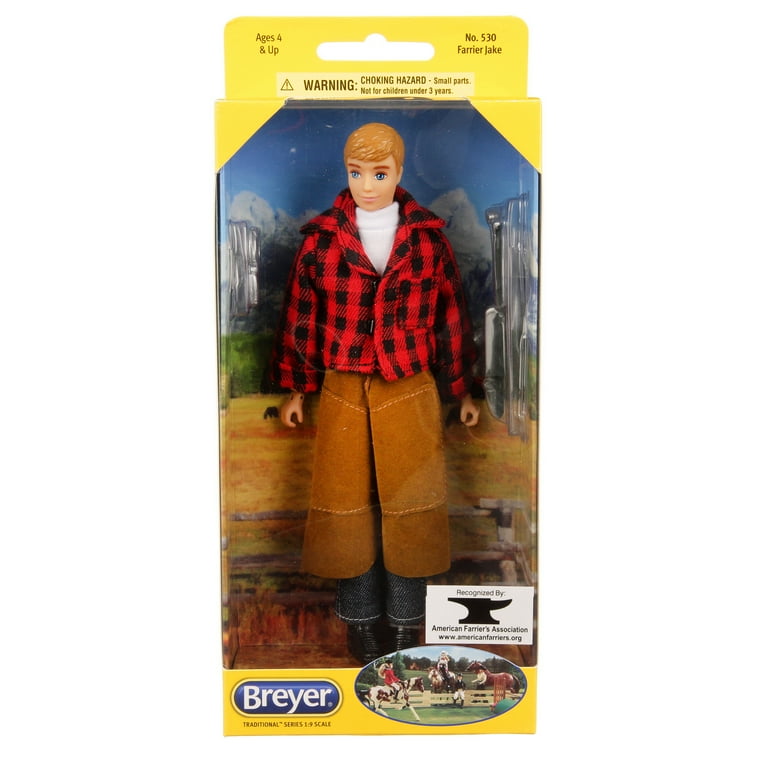The image depicts a vintage Breyer brand action figure, modeled as a farrier named Jake. The packaging, predominantly orange with accents, indicates it is suitable for ages four and up and carries a warning about small parts being a choking hazard for children under three. Additionally, the top right corner marks it as item number 530 Farrier Jake.

Jake is clad in a black and red plaid flannel shirt over a white shirt, paired with tan jeans, black boots, and a brown leather apron. The doll stands against a backdrop that appears to depict a farm scene, complete with horses, a small fence, and a farmer.

The front of the package prominently displays the Breyer logo, with the words "Traditional Series" underneath, alongside an inscription indicating a 1:9 scale. There's also a white square on the bottom right side of the packaging, stating "Recognized by the American Farriers Association," along with an unreadable website. A detailed anvil icon reinforces Jake's occupation as a farrier.

Jake is depicted with blue eyes and light brown hair, and next to him, there seems to be a set of farrier tools, although they are difficult to discern. Overall, this detailed and specialized action figure encapsulates a unique aspect of rural life, perfectly fitting the theme of traditional craftsmanship and farm maintenance.